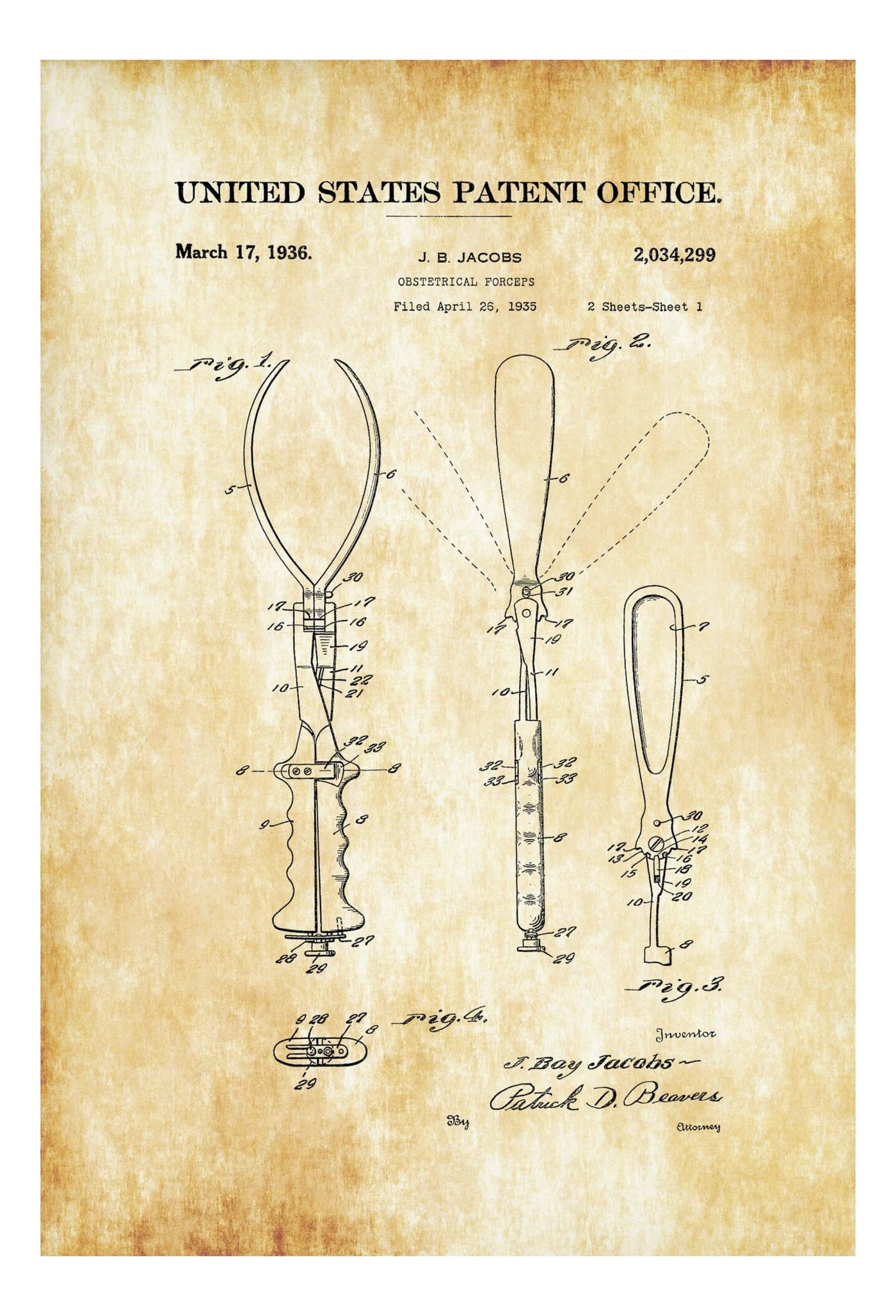This image depicts an aged, yellowed patent diagram from the United States Patent Office, dated March 17, 1936, for an invention by J.B. Jacobs, patent number 2,034,299. The paper shows evident signs of wear with large splotches of yellowing, enhancing its antique appearance. The patent drawings illustrate a detailed mechanical device, seemingly metallic and pincer-like. The primary diagram on the left reveals a clamp with two inward-curving claw-like pincers. The second drawing showcases a handle that flips out, resembling a paddle. The final illustration features an elongated bar with an oval cutout and various numbers indicating different parts. The name J. Bay Jacobs appears prominently, suggesting the inventor's identity.